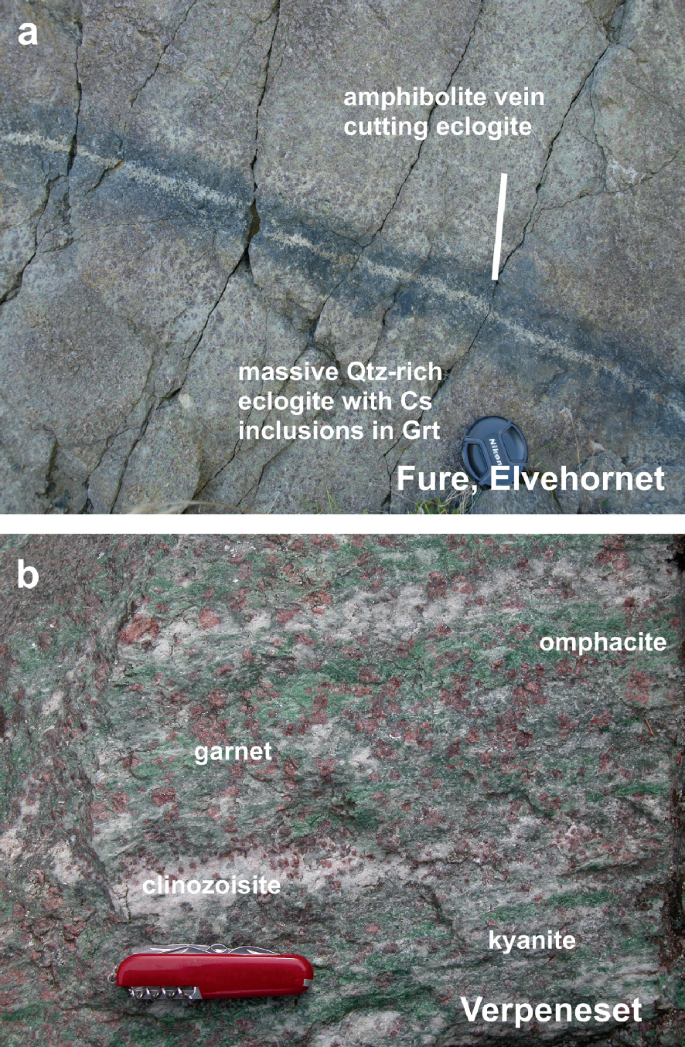The image consists of two stacked photographs labeled A and B, each depicting geological features of a rock formation. Picture A, at the top, showcases a gray rock with visible lines, some of which might be remnants of liquid flow. This image is labeled with several white annotations, describing features such as an "Amphibolite Vein Cutting Eclogite" and "Massive Quartz Rich Eclogite with CS Inclusions in GRT." Additional labels point out minerals like Omphacite, Garnet, Clinozoisite, and Kyanite, highlighting the rock’s complex mineralogy with reddish and greenish areas. There appears to be a Swiss Army knife placed on the rock for scale, and another label mentions "Verpenasit" and possibly "Fuehrer Elva Hornet." Picture B, while less detailed in description, complements A by also showing the Swiss Army knife at the bottom, reinforcing the context of fieldwork or study. Together, these images resemble textbook illustrations, potentially for educational purposes, likely documenting the geology of an area referred to as Verpanaset or Verpenasit, with a particular interest in garnet and associated minerals.